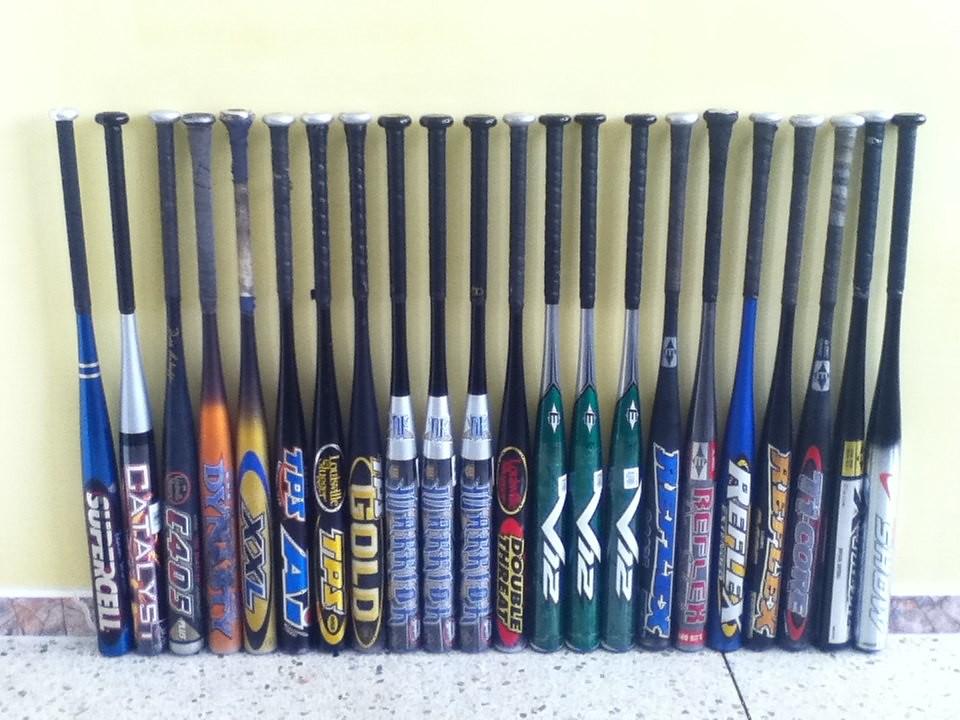The image captures a vibrant collection of around 26 aluminum baseball bats standing upright against a pale yellow wall, all lined up and touching. Each bat is made of aluminum and identical in size, yet they vary in color and brand. Starting from the left, the first bat is blue with a black handle, labeled "Supercell." Among the lineup, there are bats branded as "Catalyst," "C405," "Dynasty," "XXL," and "TPS." Notably, one bat is black with gold text reading "Gold." The next group includes three bats marked "Double Threat," followed by three green bats with white patterns labeled "V2." Subsequent bats in the row, branded "Reflex," exhibit different color schemes. The floor beneath the bats is speckled white terrazzo, adding contrast to the colorful array of bats. Some of the bats are turned in such a way that their brands are not readable, but the overall display showcases a striking variety of brands and colors, contributing to a visually engaging scene.